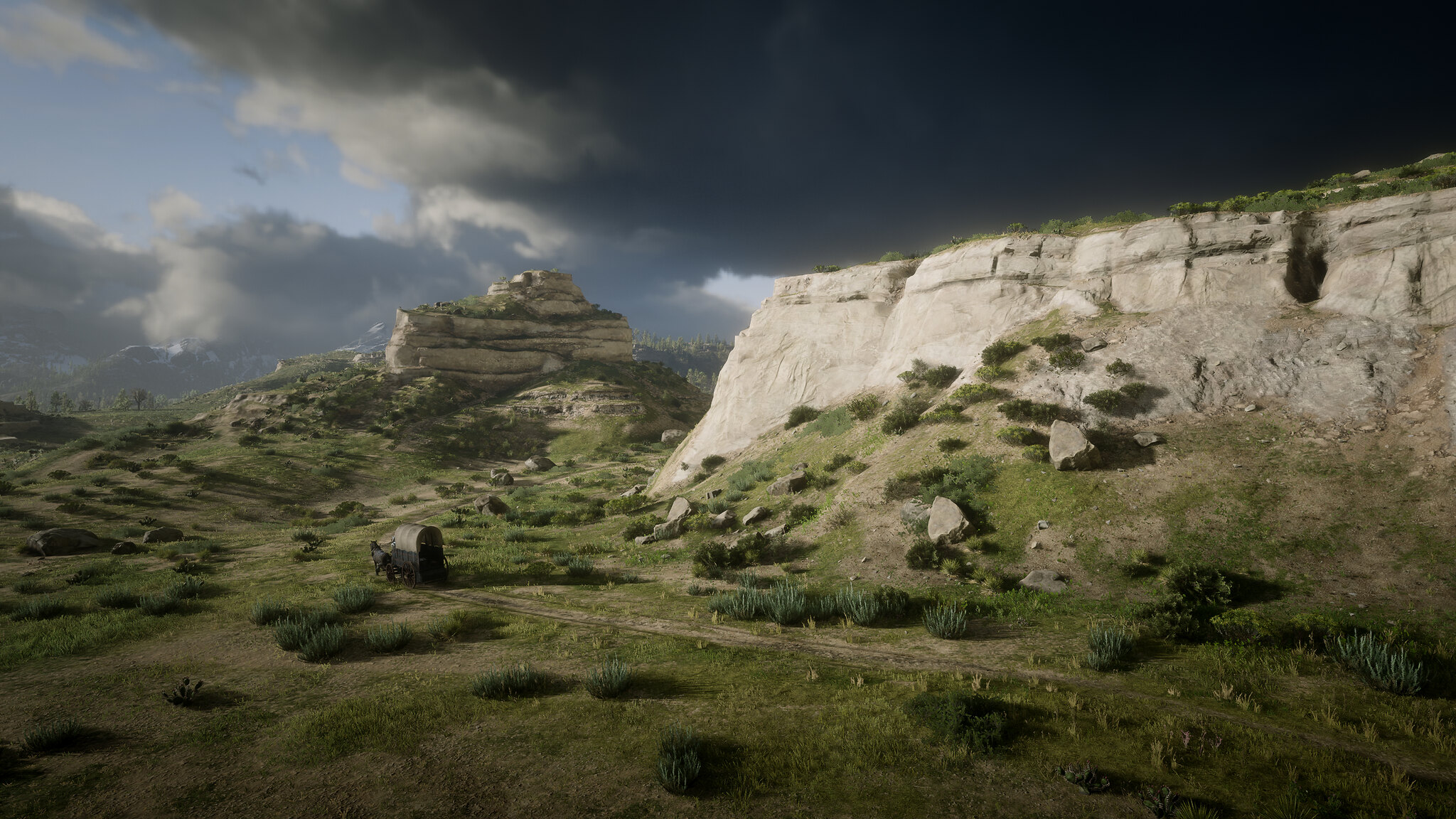The image is a highly detailed, photorealistic depiction of a vast grassy plain overlooked by rocky, angular hills and mesas. Dark, stormy clouds dominate the sky, rolling from the left with only patches of blue still visible before the entire sky becomes ominously dark to the right. In the foreground, a well-defined trail cuts across the valley, where a covered wagon drawn by dark horses is making its way towards the distant rocky hill. The wagon itself has a dark wooden base with a light top. The landscape is dotted with low grass and desert-like brush, creating a rugged and untamed environment. Flat-topped mesas with sheer, smooth rock faces and sporadic grassy spots add to the dramatic scene, hinting at the impending storm. The imaginative composition blends natural features with a touch of the surreal, giving it a realistic yet slightly hyperrealistic quality.